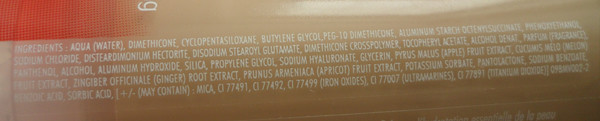This image depicts a close-up of an ingredient list on a tan-colored package. The label is horizontally rectangular, bordered by a small red or orange section on the upper left-hand side. The ingredients are written in tiny white text. Among the listed items are aqua (water), dimethicone, cyclopentasiloxane, butylene glycol, PEG-10 dimethicone, aluminum starch, sodium chloride, aluminum hydroxide, silica, propylene glycol, sodium hyaluronate, and glycerin. The text is difficult to read and some ingredients are hard to pronounce, suggesting the item could be a cosmetic product such as a gel, given the presence of silicones and glycols.